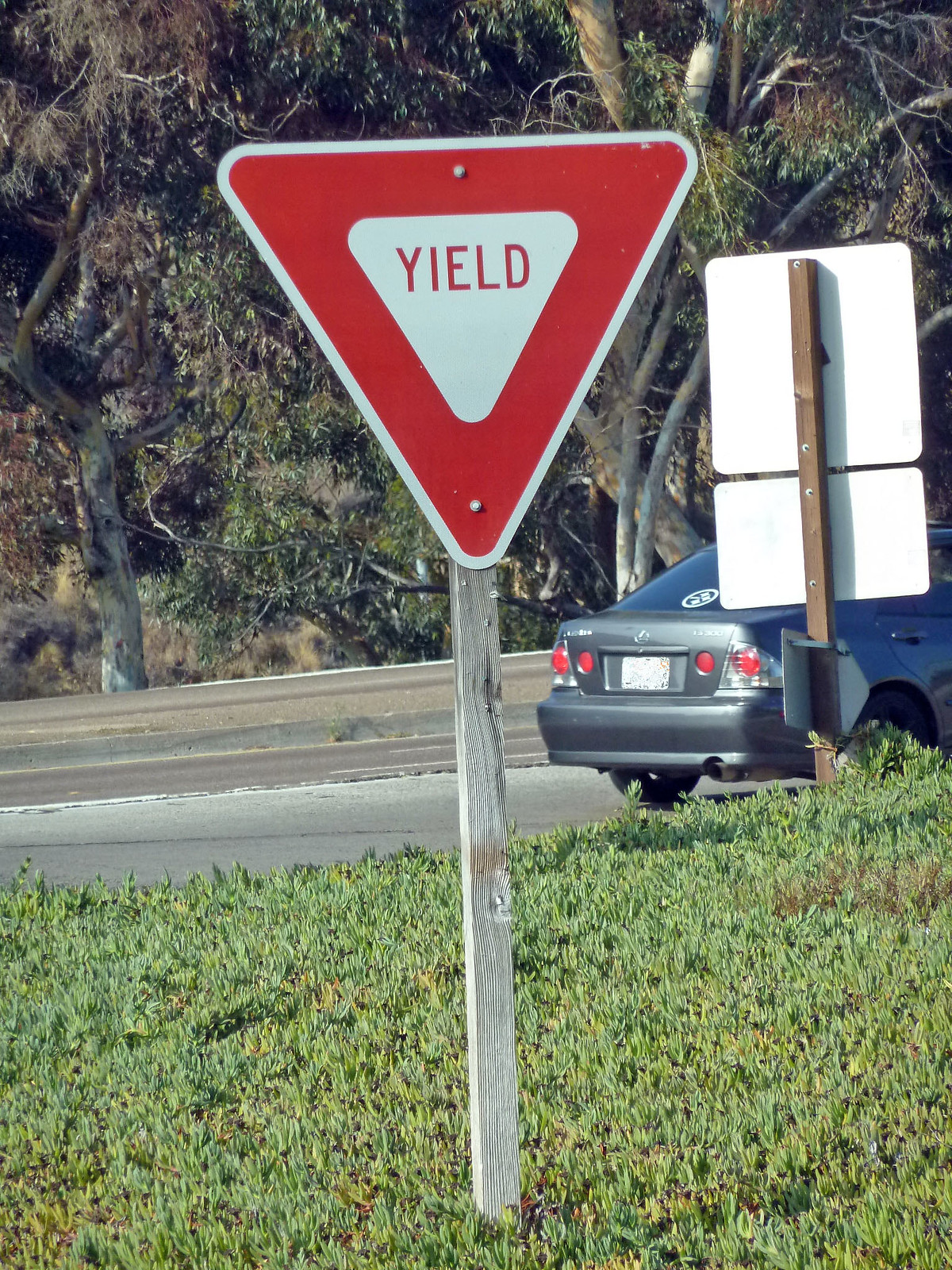The photograph captures a street scene bathed in bright daylight, emphasizing a prominent yield sign in the foreground. The yield sign, an upside-down red triangle with a rounded white border and an inset white triangle, has the word "YIELD" displayed in red capital letters in its center. The sign is mounted on an old, weathered wooden post embedded in a patch of green grass dotted with weeds. 

To the right of the yield sign, partially obscuring a view of a silver or gray car with red brake lights and a white license plate, is the back of another sign. This secondary sign comprises two white square and rectangular panels atop each other, fixed to another wooden post. The asphalt road runs horizontally through the middle of the image, its surface showing signs of wear and aging. 

In the background, a green and brown wooded area with mature trees and long green leaves frames the scene, adding a natural backdrop to the urban setting. The combination of these elements creates a vivid, detailed snapshot of a quiet street under the clear blue sky.